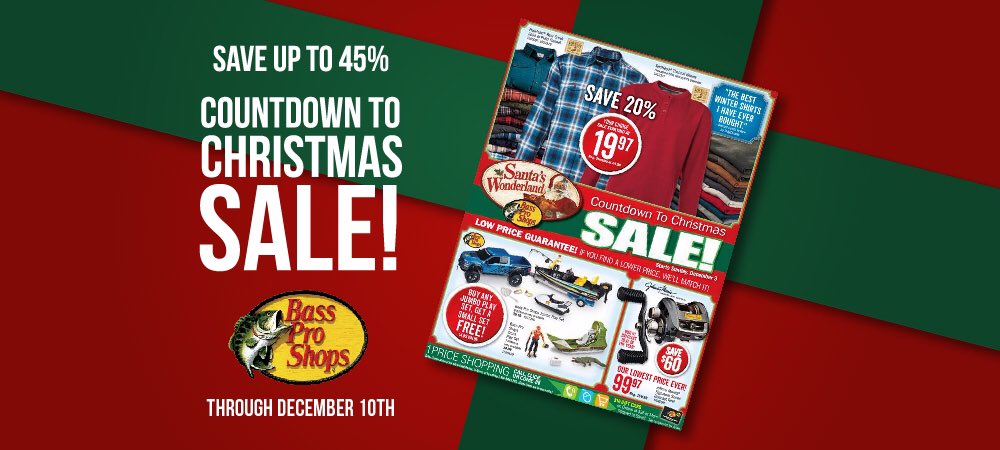The image depicts a festive promotional flyer for Bass Pro Shops featuring their "Countdown to Christmas Sale." The top of the page, adorned in red and green hues, prominently displays the bold, capitalized text "SAVE UP TO 45% - COUNTDOWN TO CHRISTMAS SALE." The Bass Pro Shops logo sits just below, encased in a yellow circle with a black outline, containing a green and white fish. The sale runs through December 10th.

Adjacent to this, a section of the flyer showcases various folded shirts, including solid colors and checkered patterns in red and white, and blue and white. These collared shirts feature three buttons and are advertised as "The best winter shirts I've ever bought," priced at $19.97 each.

Further down, the flyer highlights "Santa's Wonderland at Bass Pro Shops" with images of Santa and festive ivy surrounding the text. The "Countdown to Christmas Sale" offers a low price guarantee, promising to match any lower prices found elsewhere. A special offer is noted: "Buy any jumbo playset, get a smaller set free," illustrated by images of a car, a boat, and a doll.

To the right, a black fishing rod with matching handles is prominently displayed, advertised with a $60 discount, making the final price $99.97 – the "lowest price ever" for this item. The bottom of the page emphasizes the convenience of "One Price Shopping."